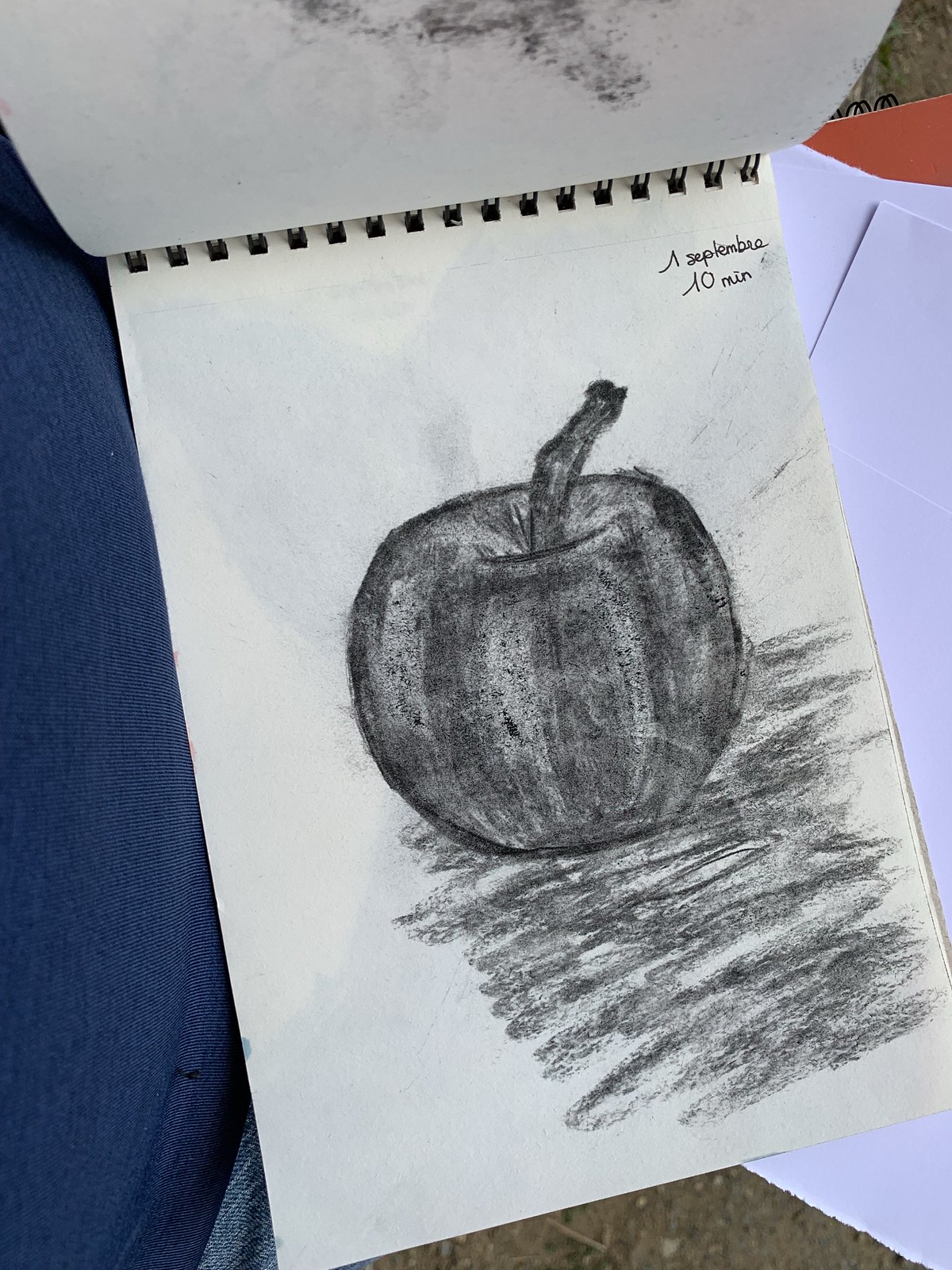A photograph captures the inside of an artist's sketchbook. The sketchbook features white paper and a black ring-bound edge along the top. Drawn in black charcoal, the artwork depicts an apple with a pronounced stem, shaded heavily in dark black tones. The charcoal has smudged onto the page above, adding to the raw aesthetic. Accompanying the apple is a shadow or ground area made with charcoal beneath it, providing depth. The sketchbook rests next to someone's leg clad in blue jeans. In the background, additional sheets of paper and another notebook add context to the scene. Handwritten notes are visible at the top of the sketchbook page, possibly in another language, with the words "September" and "ten minutes" discernible.